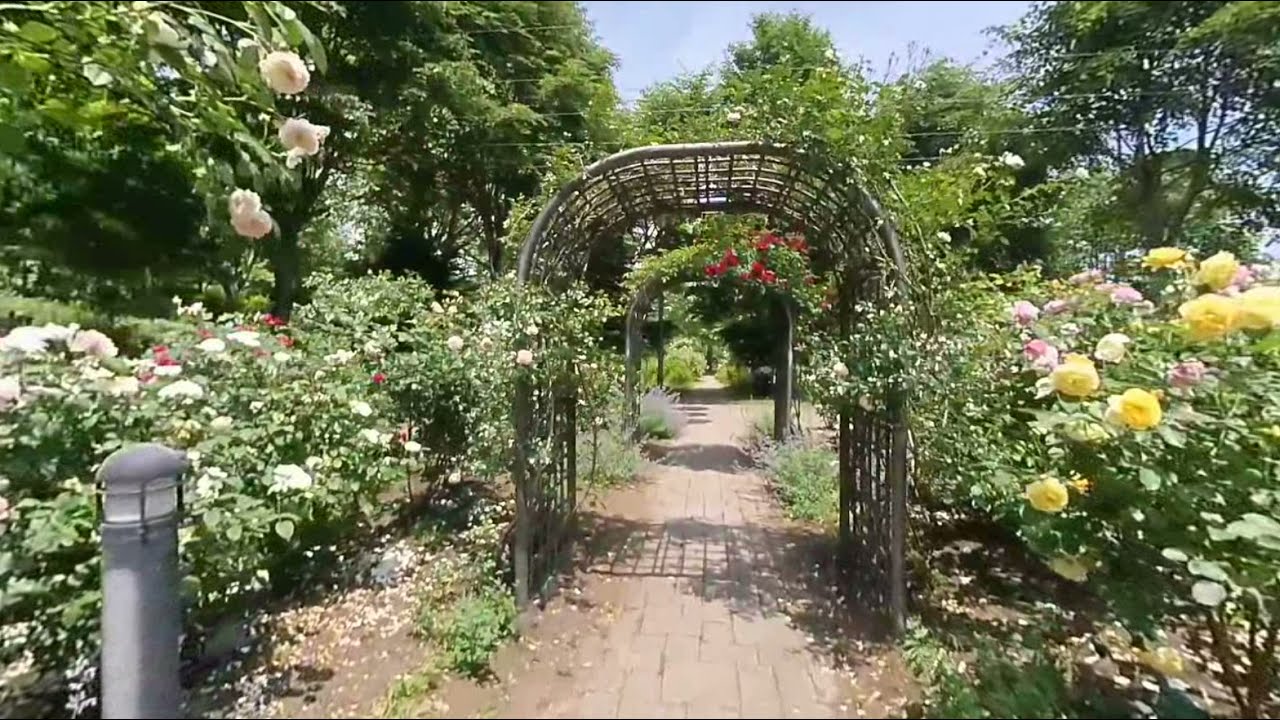This stunning photograph captures the entrance of a vibrant outdoor garden under a sunny, blue sky speckled with white clouds. The centerpiece is a narrow pathway, made of light beige and red rectangular bricks, directly leading into the garden. Along this inviting path, two elegant, rectangular garden arbors with curved tops and wooden structures are adorned with climbing vines and blooming roses, creating a picturesque tunnel effect.

On the left side of the path, a diverse array of flowers includes white, red, and dark pink roses, with some peach-colored roses hanging from a flowering tree in the top left corner. The left side also features a light stand. The right side of the path is equally colorful with bright yellow and shades of light and dark pink roses scattered among various plants.

In the background, numerous trees extend towards the horizon, and some wires subtly cross the top portion of the image, adding a touch of modern contrast to the natural beauty. The path enticingly leads further into a larger garden, hinting at more floral splendor beyond the visible scene.